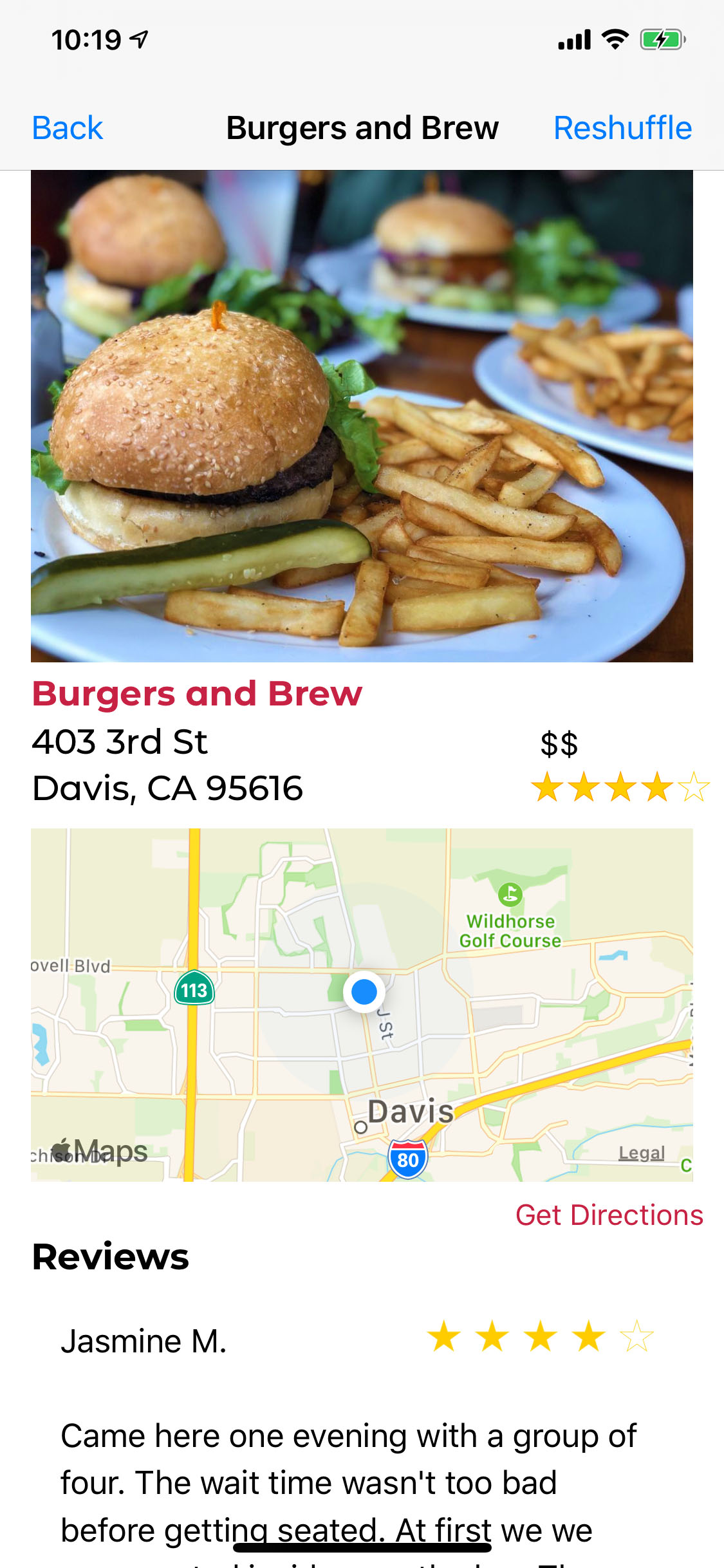A smartphone screen displays a Yelp search for "Burgers and Brew," captured at 10:19. The interface includes a back button on the left and a "Reshuffle" option in blue on the right. The search term "Burgers and Brew" is prominently displayed at the top. Below, there’s an appetizing image of a plate featuring a juicy burger, crispy fries, and a pickle. The burger is garnished with fresh green vegetables. 

Underneath the image, in bold red text, it reads "Burgers and Brew," followed by the address "403 3rd Street, Davis, CA 95616," accompanied by a four-star rating. Further down, a map illustrates the location. Below the map, a review from user Jasmine M., who gave a four-star rating, starts with: "Came over one evening with a group of four. The wait time wasn't too bad before getting seated. At first we…" The review is cut off at this point by the edge of the screenshot.